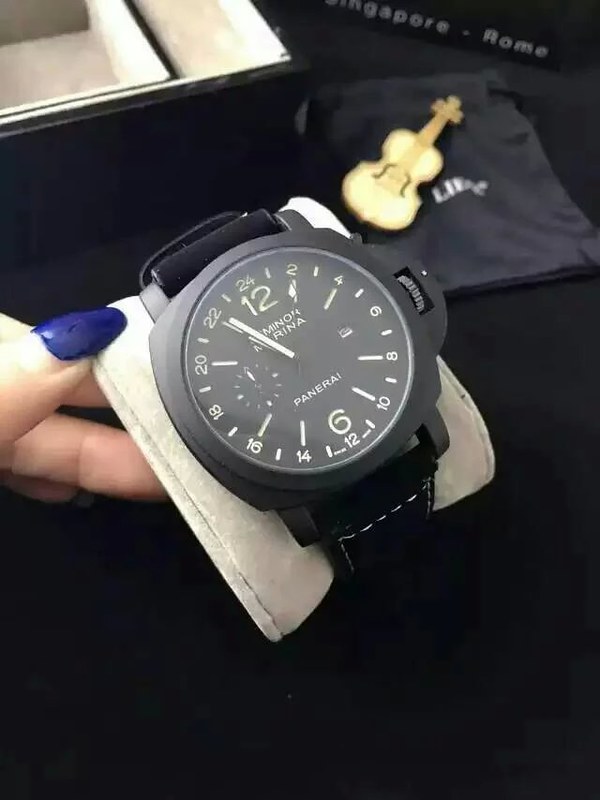This image features a sophisticated black wristwatch elegantly displayed on an off-white wrist-shaped stand, commonly used in jewelry stores. The stand is a subtle gray color, providing a neutral backdrop that accentuates the watch. The watch itself has a black case and a white clock face. Notably, it has a textured gray dial located to the right, encased in black, with a tactile grating that allows for easy adjustment.

The clock face of the watch prominently displays the numbers 12 and 6, with minimalist dashes replacing the other hour markers. Surrounding these dashes are numbers that denote military time: 24, 2, 4, 6, and 8. Above the 6 o'clock position, the brand name "Panerai" is written in elegant white letters. The text below the 12 o'clock position is partially obscured by the clock's white hands.

To the right of the watch, there is a small, intricately detailed model of a gold violin, positioned atop what appears to be a black bag featuring unreadable white text. A human hand, adorned with blue artificial fingernails, holds the display cylinder, adding a touch of personality to the image. The background is predominantly black, with some color and letter-like objects faintly visible near the top edge of the frame.